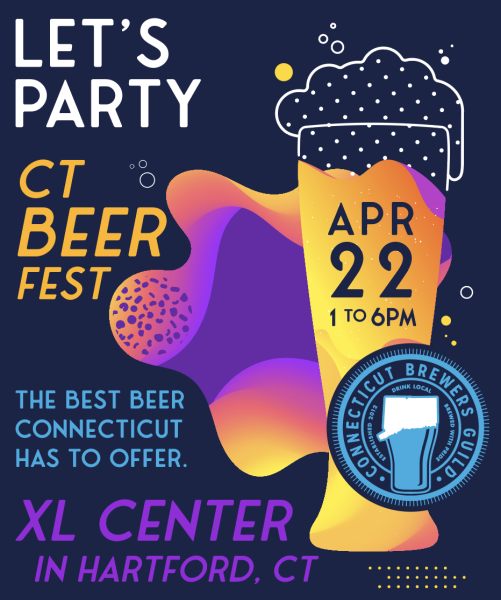The image is a vibrant, detailed poster for an upcoming event, set against a dark blue background. At the top left, bold white text announces "Let's Party," followed below by cheerful yellow text stating "CT Beer Fest." Moving down the left side, light blue text declares, "The Best Beer Connecticut Has to Offer," and beneath it, bold purple text specifies the venue, "XL Center in Hartford, CT."

On the right side, there is a striking, computer-drawn beer glass, filled with an orange-yellow liquid and topped with frothy foam. Inside the top of the glass, dark blue text marks the event date and time: "APR 22 1-6 PM." Just beneath the glass, a small, patch-like blue, white, and black label prominently features the Connecticut Brewers Guild logo and the slogan "Drink Local." The interplay of colors like blue, purple, orange, and yellow throughout the poster creates an engaging and festive atmosphere.